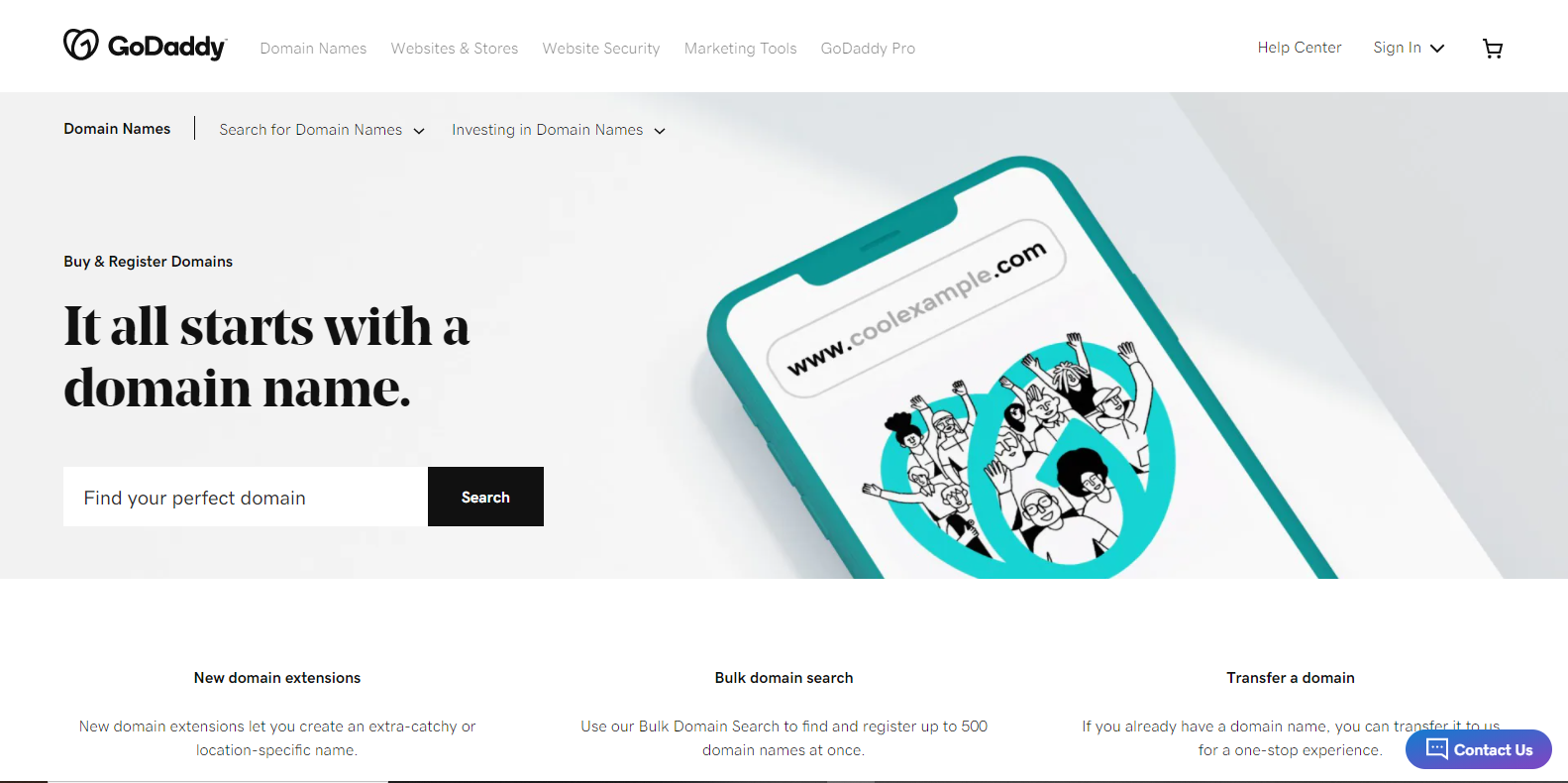This image is a detailed screenshot of the GoDaddy homepage, presented in landscape orientation. Starting from the top left corner, the GoDaddy logo is prominently displayed in black lettering, accompanied by the GoDaddy icon. Spread across the top are various navigation tabs in light grey: Domain Names, Websites & Stores, Website Security, Marketing Tools, and GoDaddy Pro. On the right-hand side, the page features a Help Center link, a 'Sign In' option with a dropdown arrow, and a cart icon.

Dominating the middle of the image is a large grey banner, which reads "Buy and Register Domains." The tagline beneath it states, "It all starts with a domain name," followed by a search bar with placeholder text, "Find your perfect domain." Adjacent to the search bar is a black search button labeled "Search" in white text. The graphic within this grey banner is a stylized illustration of a mobile phone. The phone, which is green, displays "www.coolexample.com" on its white screen, flanked by a turquoise heart and outlined, smiling cartoon figures with their hands raised, demonstrating a sample website created using GoDaddy.

Beneath this main grey box, the page elaborates on services offered:
- On the left side, "New Domain Extensions" highlights the benefit of creating catchy or location-specific domain names with new extensions.
- In the center, "Bulk Domain Search" encourages users to find and register up to 500 domain names at once.
- On the right side, "Transfer a Domain" invites users to transfer their existing domain names to GoDaddy for a seamless experience, accompanied by a blue button labeled "Contact Us" in white text with a speech bubble icon.

Additionally, within the top grey banner to the left, terms like "Domain Names," "Search for Domain Names," and "Investing in Domain Names" are featured, guiding users to specialized areas for domain-related services.